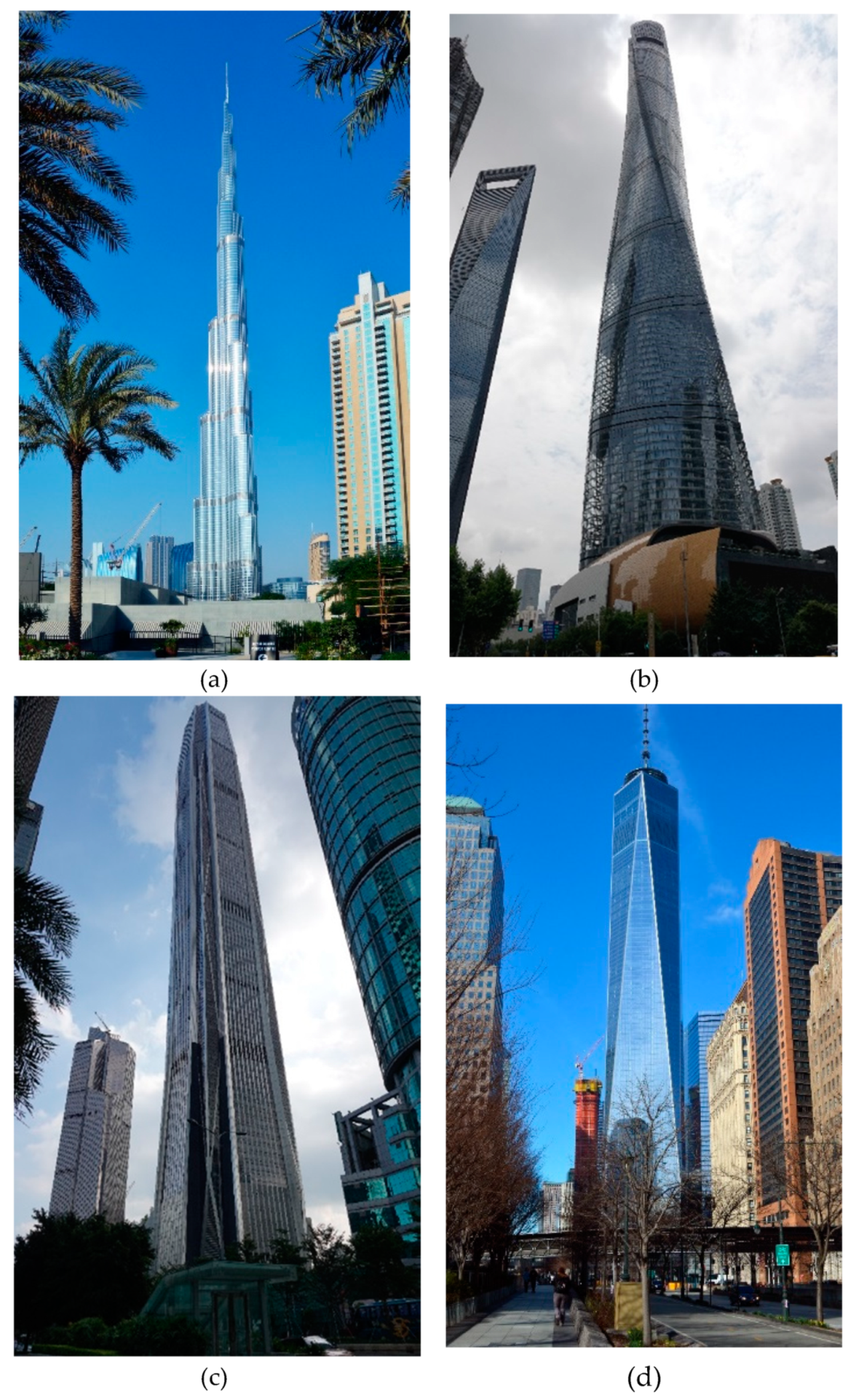This collage features four distinct photographs of skyscrapers, labeled A through D, arranged in a square with two images on top and two on the bottom. Picture A showcases a towering skyscraper with a prominent spire, surrounded by palm trees, suggesting a beachy locale, possibly Miami. Picture B, positioned to the right of A, captures a very tall, cylindrical skyscraper with a spiral design, set against a cloudy sky, with a straight, tall building visible to its left. Below A, Picture C displays a thin, rectangular skyscraper with a clean, squared-off appearance, accompanied by smaller buildings and palm trees. Finally, Picture D, located to the right of C, features a large, rectangular skyscraper with a spire or antenna at the top, flanked by shorter buildings, and bare trees visible in the foreground. All buildings are distinct in their architecture, emphasizing their grand scale and unique designs.